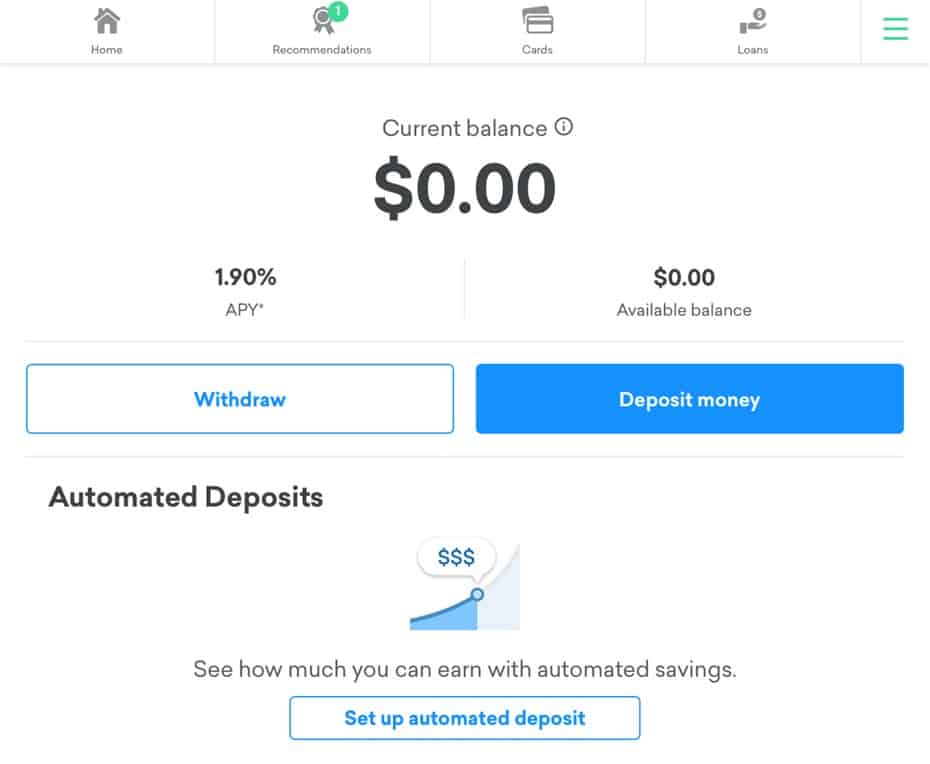The image features a digital financial dashboard set against a white background. At the top, there's an illustration of a house, accompanied by the word "home" beneath it. Adjacent to this is a ribbon labeled "Recommendations," followed by a green circle with a white number "1" inside it.

In the center, there's an image showing the front and back of a credit card, with the label "Cards." Nearby, a hand is extended, pointing to the right, towards a circle containing a white dollar sign, labeled "Loans."

On the right side, green bars are displayed alongside text centered around debt. It includes a section titled "Current Balance," next to a circled information icon ("i"). The current balance is shown in black, which is zero, suggesting that there is no outstanding debt. The Annual Percentage Rate (APR) is indicated as 1.9%, with zero credit available. Below this is a white rectangular button with blue text that reads "Withdraw," and an inverse button on the right stating "Deposit Money."

Towards the bottom left, the dashboard highlights "Automated Deposits," featuring a bar graph with ascending dollar signs, emphasizing the potential for savings. The section includes a call to action: "See how much you can earn with automated savings." Below it, there is a white button with blue text that says "Set Up Automated Deposit."

Overall, this detailed financial dashboard visually organizes various personal finance elements, making it easy to track recommendations, card information, loans, current balance, and savings automation options.